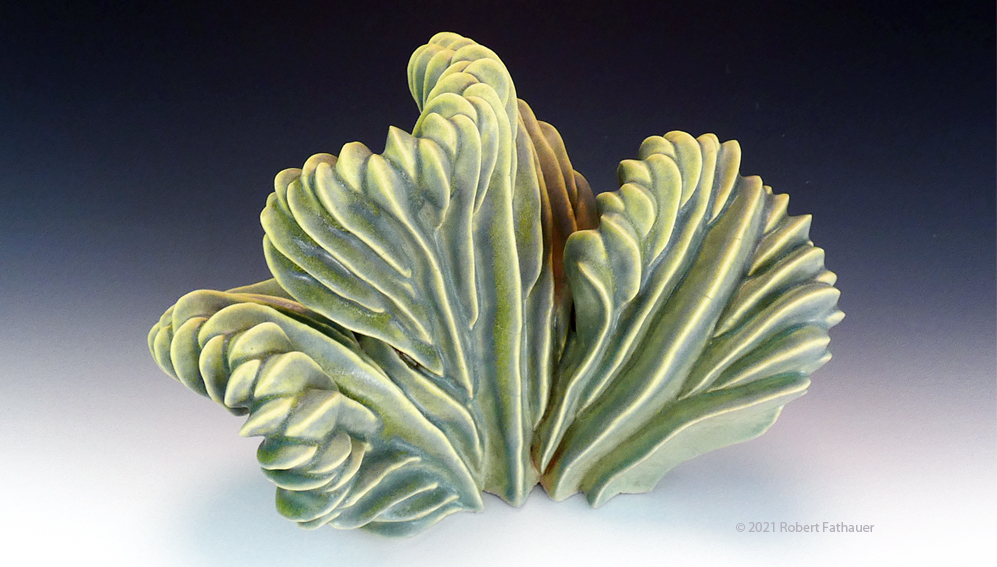The image showcases a digital art print or painting featuring what appears to be an exotic plant with three leaves. The background transitions smoothly from black at the top to dark blue, light blue, and finally white at the bottom, creating an ombre effect that accentuates the plant. The leaves, varying in shades of green, exhibit a characteristically textured and ridged appearance. The leaf on the bottom left is positioned on its side, the central leaf stands upright with a curve at the top, and the third leaf shoots out from behind the middle one, curving inward. Each leaf has sharp, irregular edges reminiscent of claws, and the ridges create intricate shadow patterns and white streaks along their lengths. A touch of brown on the central leaf suggests natural imperfections or decay. In the bottom right corner of the artwork, the signature reads © 2021 Robert Fathauer, verifying the artist's identity.